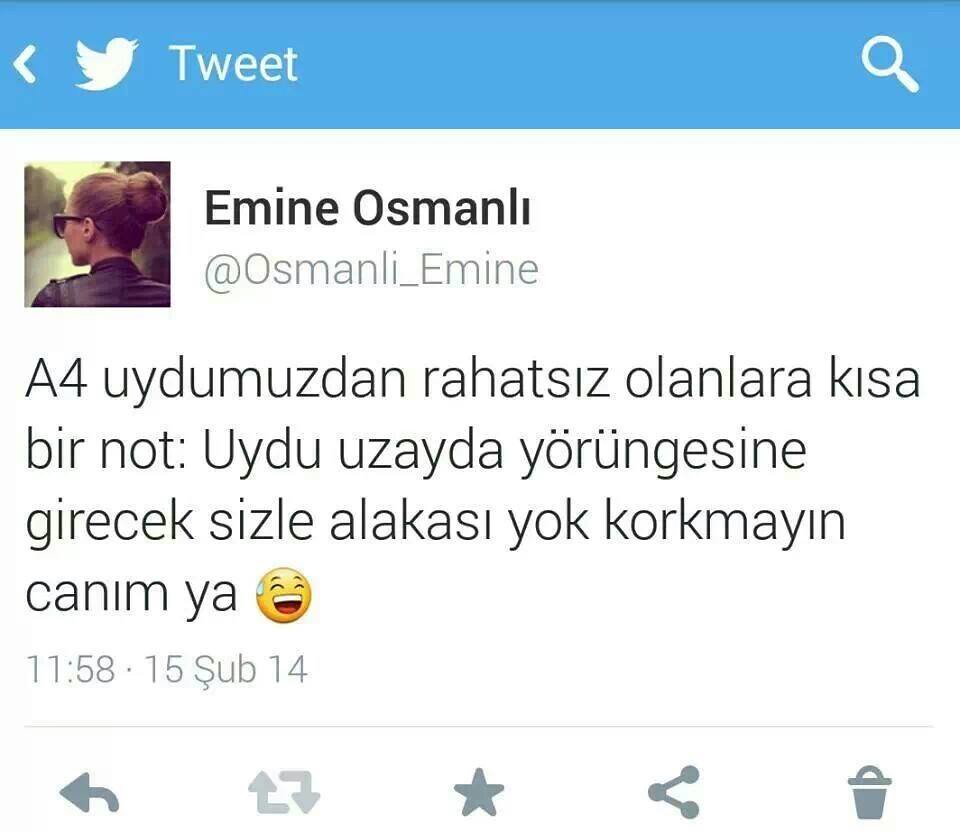The image shows a screenshot of a tweet with a baby blue border at the top, featuring the white Twitter bird icon, the word "Tweet," and a search magnifying glass in the upper right corner. The profile picture belongs to a woman with blonde hair in a bun, wearing sunglasses, and looking to the left, dressed in a black shirt. Her username is displayed as "Emine Osmanli," and her handle is @Osmanli_Emine. The tweet itself is written in a foreign language and includes an emoji of a smiling face with a sweat drop. The timestamp next to the tweet reads 11:58, 15 Sep 14. Below the tweet text, there are standard Twitter navigation icons for sharing, trashing, and starring.